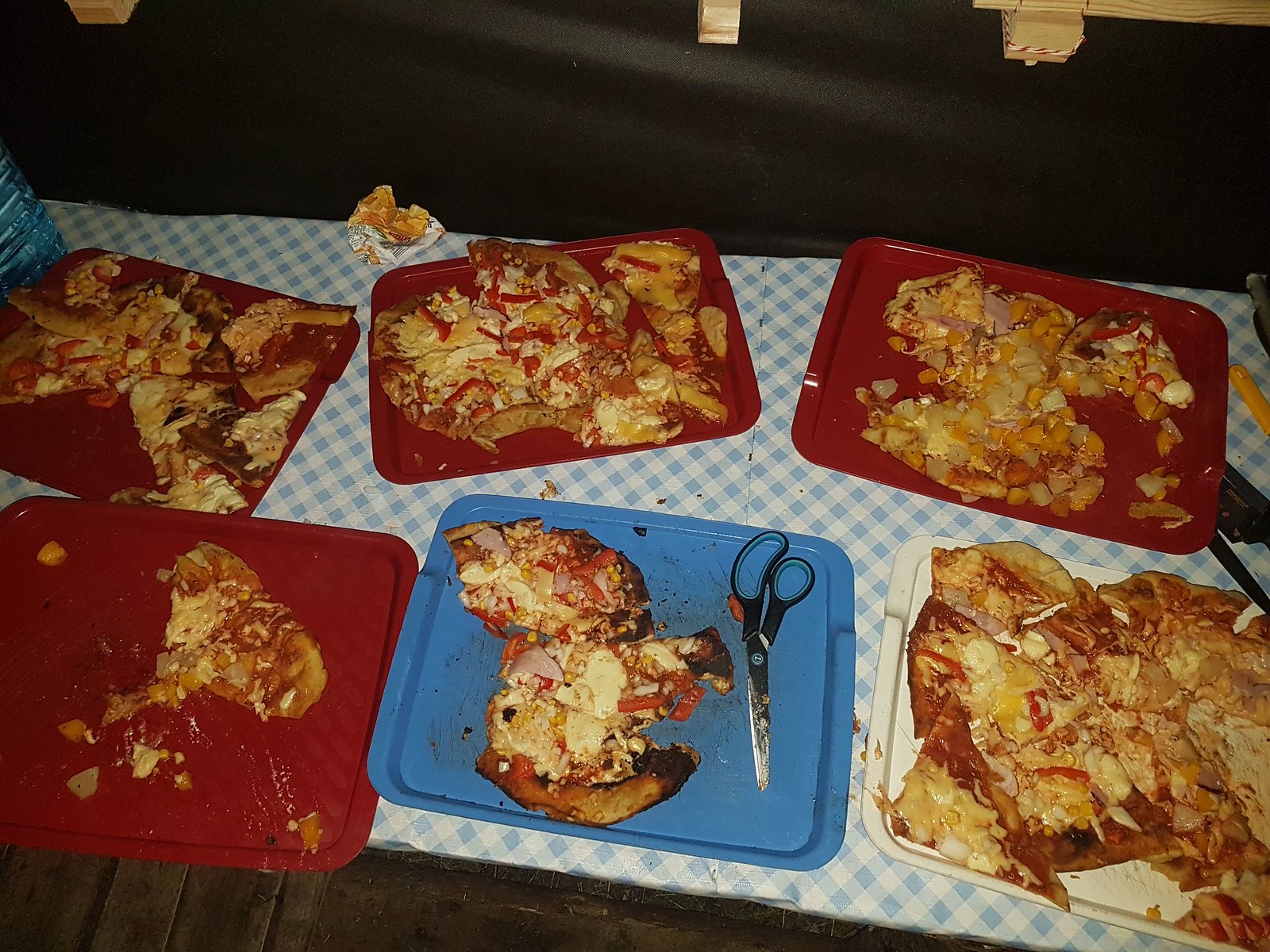The image captures a chaotic scene of six rectangular lunch trays on a country-style blue and white gingham tablecloth. Arranged in two rows of three, the top row features three red trays, while the bottom row consists of a red tray, a blue tray with a pair of closed scissors with black handles, and a white tray. Each tray holds remnants of homemade pizza that has been crudely cut into irregular shapes, likely with the scissors present. The pizza varies in appearance; some pieces are burnt, others soggy, with toppings and sauce smeared across the trays. In addition to pizza, a mixture of fruits including peaches, pineapples, and possibly grapes are scattered on one of the red trays, adding to the chaotic display. Overall, the food presents a very messy and unappetizing appearance.